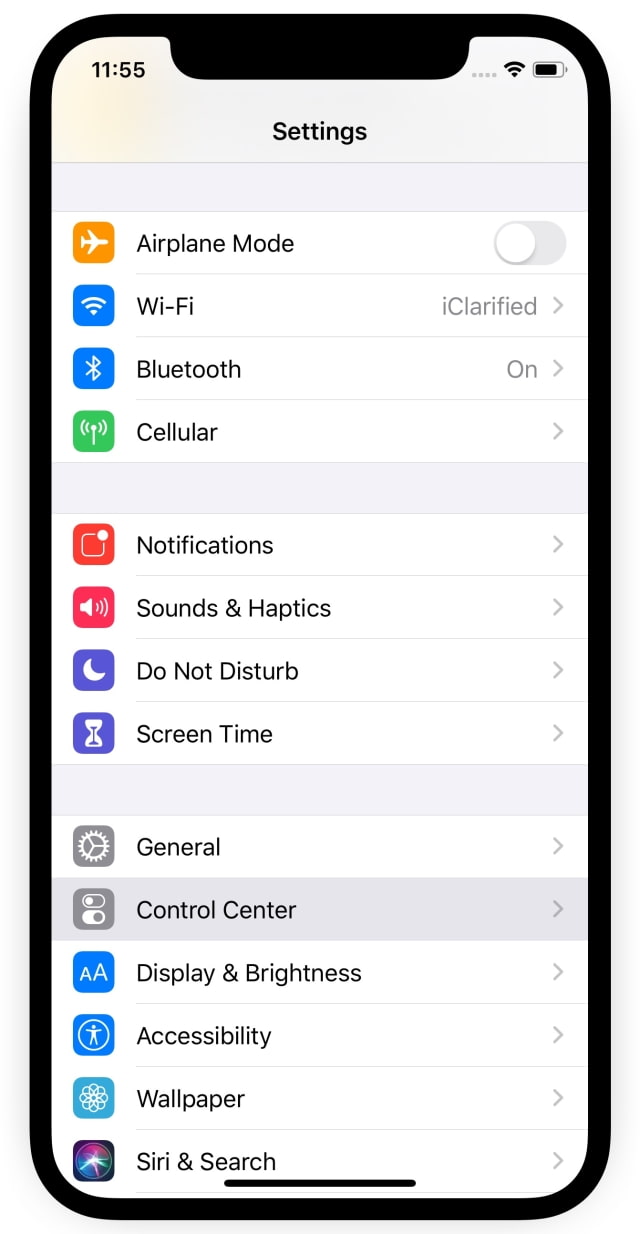The image depicts the settings menu on a cell phone with the time displayed at 11:55 in the upper left corner. Adjacent to the time, there is a full Wi-Fi icon and a battery icon. The settings menu is organized into various categories: 

1. **Connectivity Options**:
   - **Airplane Mode**: Switchable via a button on the far right.
   - **Wi-Fi**: Indicated as active with a clarifying note and an arrow to access subcategories.
   - **Bluetooth**: Currently turned on.
   - **Cellular**.

2. **Notifications and Sound**:
   - **Notifications**: 
   - **Sounds and Haptics**.
   - **Do Not Disturb**.
   - **Screen Time**: This section is separated by a thick gray line.

3. **General Settings**:
   - **General**: Separated by another gray line.
   - **Control Center**.
   - **Display & Brightness**.
   - **Accessibility**.
   - **Wallpaper**.
   - **Siri & Search**.

Each setting category is accompanied by a relevant icon, providing a visual representation of the function. The layout features various horizontal gray lines to compartmentalize different settings sections clearly.